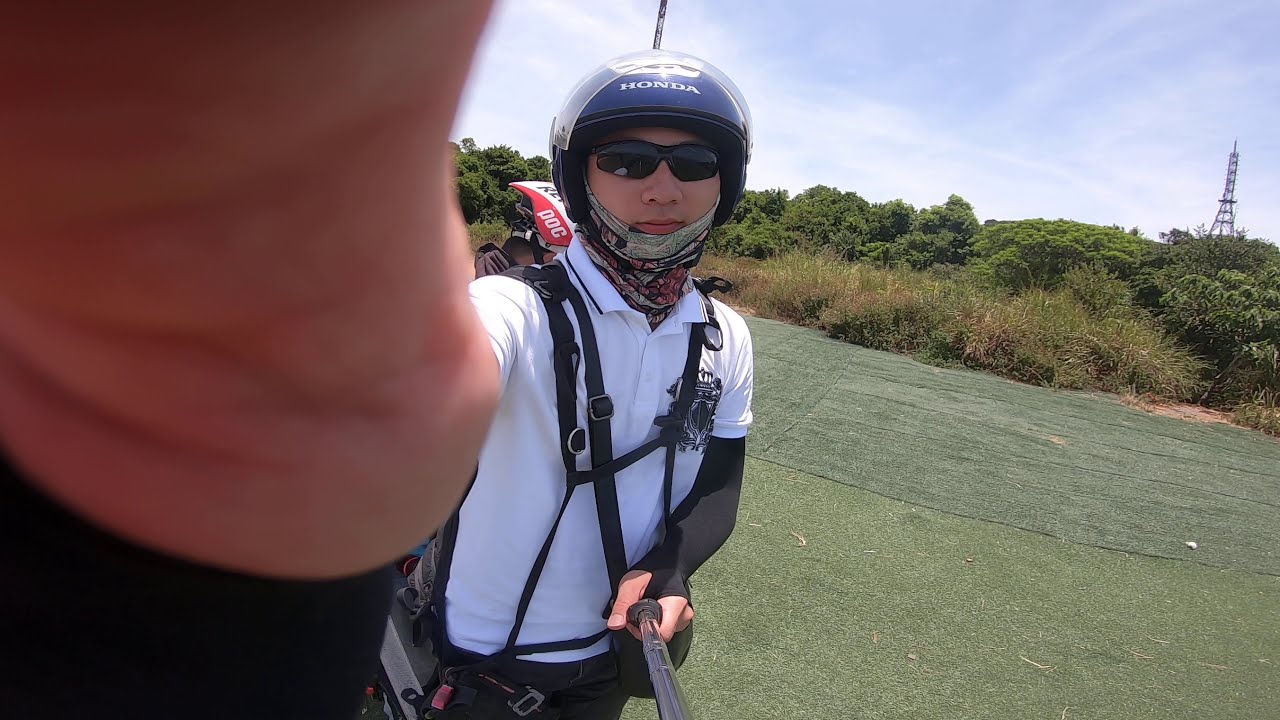This image is an outdoor scene, capturing a person standing directly in front of the camera in a grassy field. Part of the camera is obstructed by what appears to be a flesh-colored finger over the upper left-hand corner of the screen. The central focus is a Caucasian man wearing a blue and white helmet with the text "Honda" on it. The helmet features a clear visor over the top. The man is also sporting dark sunglasses and a neck gaiter or bandana under his chin. He is dressed in a white, short-sleeved polo shirt with a logo on the left breast and is wearing a black-colored harness over his shoulders and chest. The man appears to be holding a selfie stick, which is partially visible. 

In the background, extending towards the upper right-hand corner, there's a light blue sky adorned with wispy white clouds. A tall tower is noticeable near the top right of the image, set against dense trees and bushes with lush green leaves. To the right and behind the main subject is another person wearing a red and white helmet. The scene encompasses a large, flat expanse of green grass, with some areas slightly sloping, contributing to the picturesque outdoor setting.